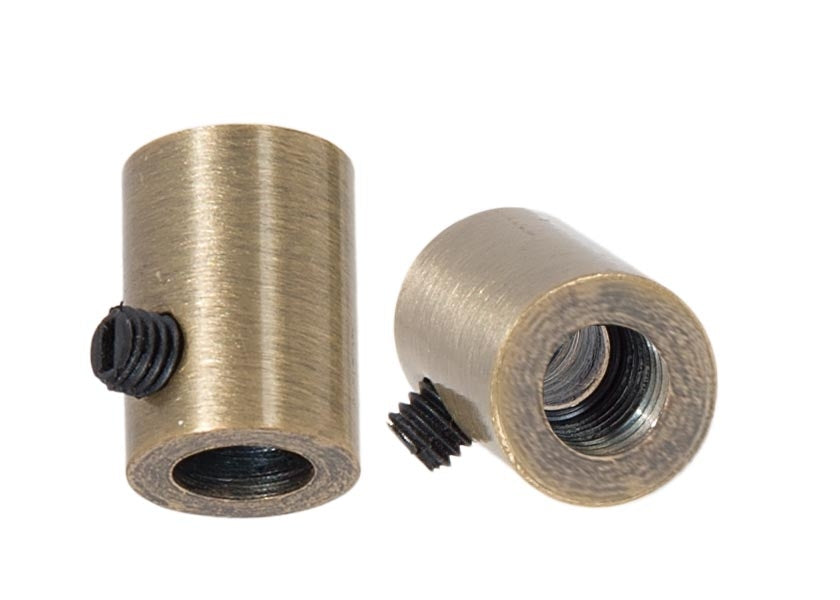This color photograph depicts two cylindrical objects made of brushed silver metal, displayed from different angles. Both cylinders are similar in size, with one standing upright at a slight tilt and the other laying horizontally. Each cylinder features a small, screw-shaped, ribbed valve protruding from the side. The exterior of the cylinders has a distinctive brushed texture. An interior view of the cylinders reveals screw threading that runs almost the entire length. The exact purpose of these metallic objects remains unclear, though they could serve as components for mechanical or electrical applications. No text, people, animals, or structures are present in the image, leaving the location and context of the photograph undetermined.